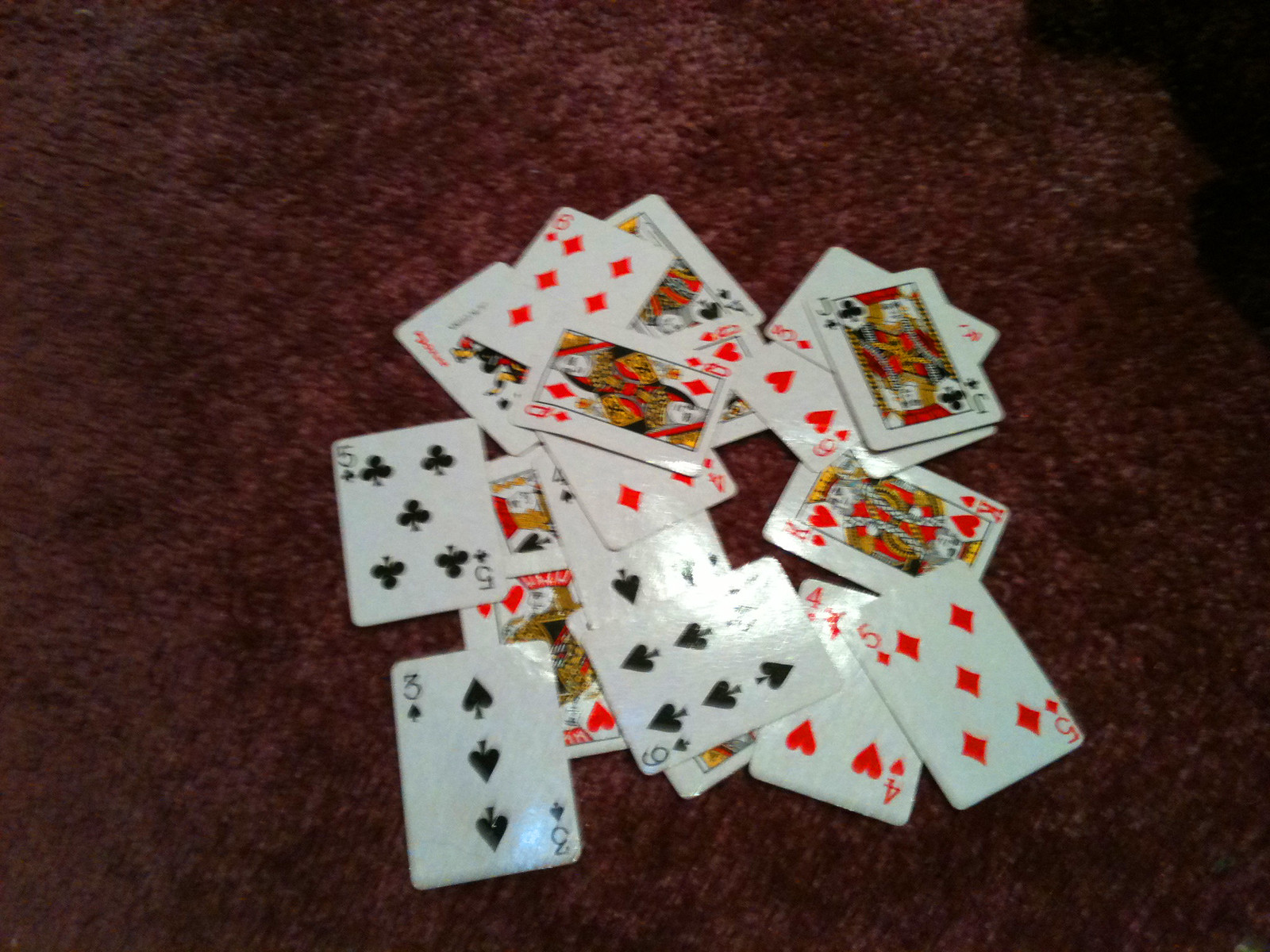This photograph showcases an array of playing cards displayed face up on a reddish-brown carpet. The glossy cards, which appear to be about fifteen in number, are not from a complete deck. Each card is clearly visible and appears to have a treated finish that enhances their sheen. Notable cards in the arrangement include the Queen of Hearts, the Jack of Spades, and various numbered cards such as multiples of fives and fours. 

In the bottom left corner, there's a number three, with a number five positioned to its right. Directly above the three is another five. Centrally located in this spread is the Queen of Diamonds, beneath which the Six of Spades is positioned at the top. To the right of the Six of Spades is the Jack of Clubs. A Joker card is slyly peeking out from beneath the Queen of Diamonds, adding a playful element to the display. The photograph is framed slightly above and to the left of the cards, capturing the textured backdrop of the carpet and creating a warm contrast to the glossy cards.